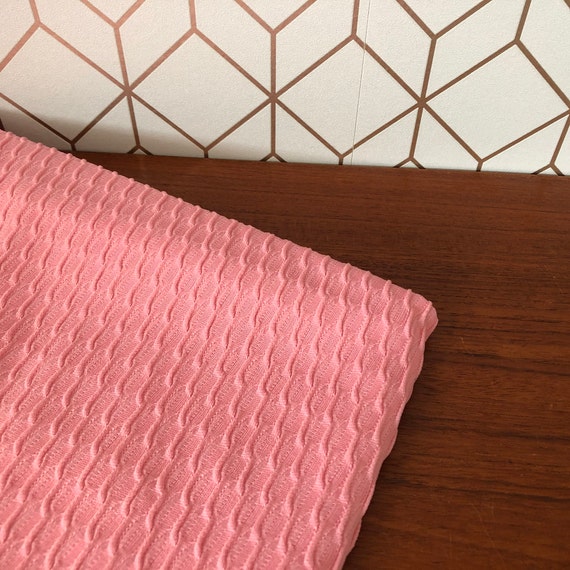The image captures an indoor setting in a photographic style, predominantly focusing on a dark, hardwood-like surface. The surface is likely a table or counter with visible scratches in the bottom right corner. On top of this surface lies a folded, light pink fabric featuring a honeycomb or interlocked link design, giving it an embossed, quilt-like appearance. The fabric could be a towel or a thin blanket with a slight peach hue. The table or counter abuts a white tiled wall, adorned with geometric patterns in brown or copper tones, enhancing the scene's intricate texture and color contrast.